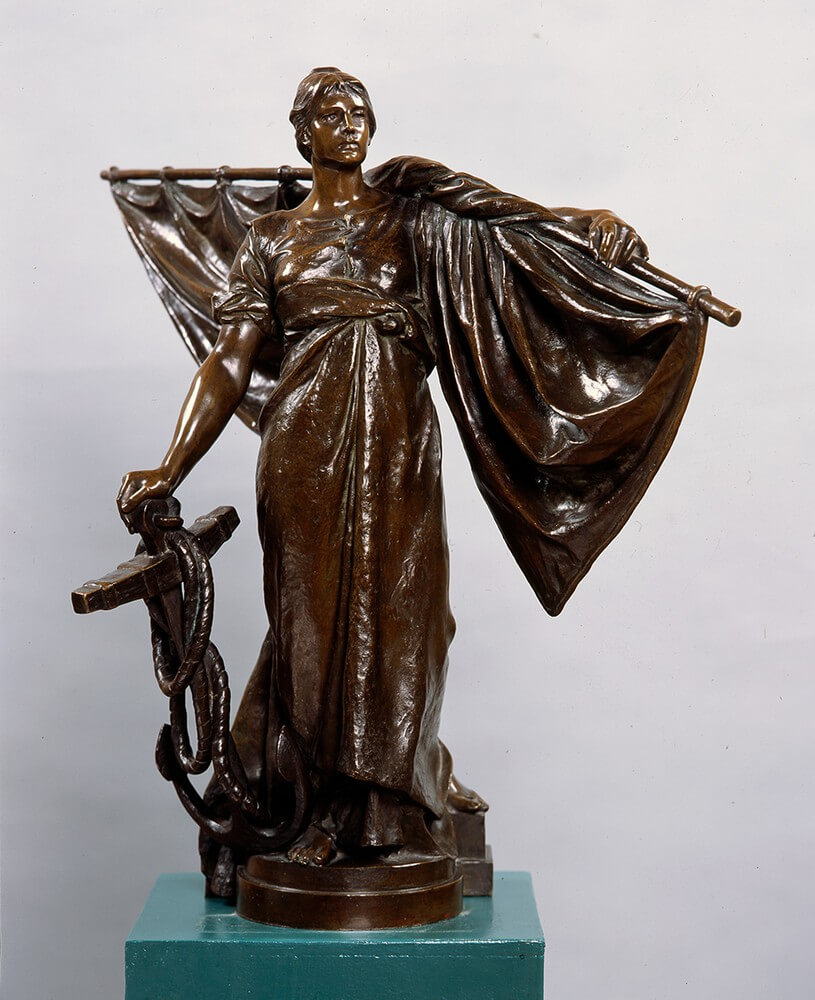The image showcases a striking bronze sculpture of a woman, standing poised on a square teal podium. The sculpture is a dark brown color with a shiny finish. The woman is elegantly clad in a long dress that flows almost down to her toes, featuring short sleeves and a neckline that hints at her shoulders and chest. Her hair is short, parted in the center, covering her ears and giving her a dignified, confident appearance.

In her right hand, she firmly holds a large, old-fashioned ship's anchor, with a rope meticulously wrapped around it, resting next to her legs. The anchor's design is classic, curving upward with hooks at the bottom. Over her left shoulder, she effortlessly carries a pole that supports a sail-like fabric draped around it. The details of the folds in the fabric are intricately captured, adding to the nautical theme of the piece.

The woman's neutral but strong facial expression, combined with her regal posture, suggests a patron saint of sailors, exuding a sense of firmness and strength. The white wall in the background provides a subtle gradient of shadow, further highlighting the sculpture's impressive and detailed craftsmanship.